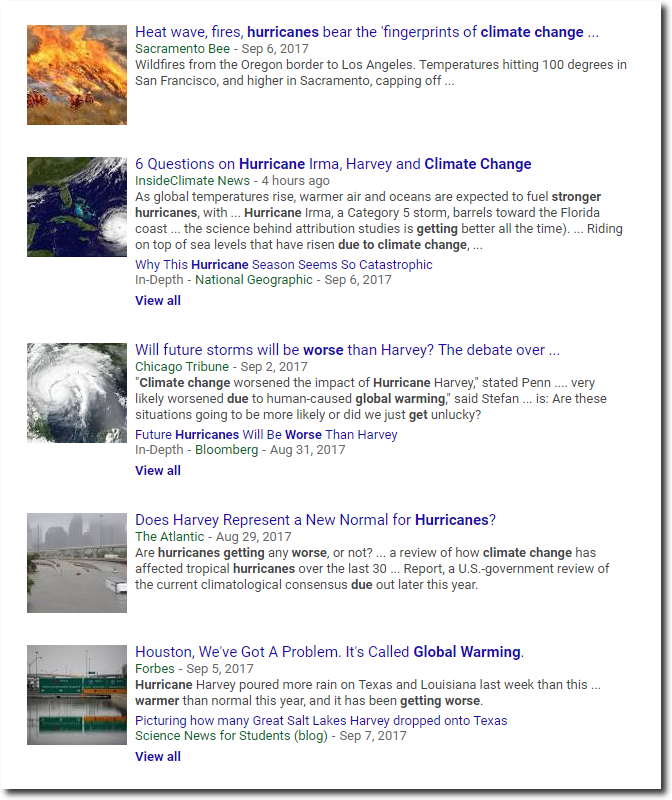A screenshot depicts a news search results page focused on climate change, characterized by a white background and black text, with hyperlinks appearing in blue. Encased in a subtle outline with a drop shadow, this interface is set against another white backdrop. The page lists five distinct articles related to various climate change events, each accompanied by corresponding imagery:

1. "Heat waves, fires, hurricanes bear the fingerprint of climate change" - Sacramento Bee. This link is paired with a photo of firefighters battling a wildfire.
2. "Six questions on Hurricane Irma, Harvey, and climate change" - Inside Climate News.
3. "Future storms will be worse than Harvey" - Chicago Tribune. The text discusses ongoing debates about the increasing severity of hurricanes.
4. "Does Harvey represent a new normal for hurricanes?" - The Atlantic. This article is illustrated with satellite images tracking the hurricanes.
5. "Houston, we've got a problem: It's called global warming" - Forbes. Another satellite photo displays the extent of hurricane activity and damages, alongside pictures depicting flooding in different areas.